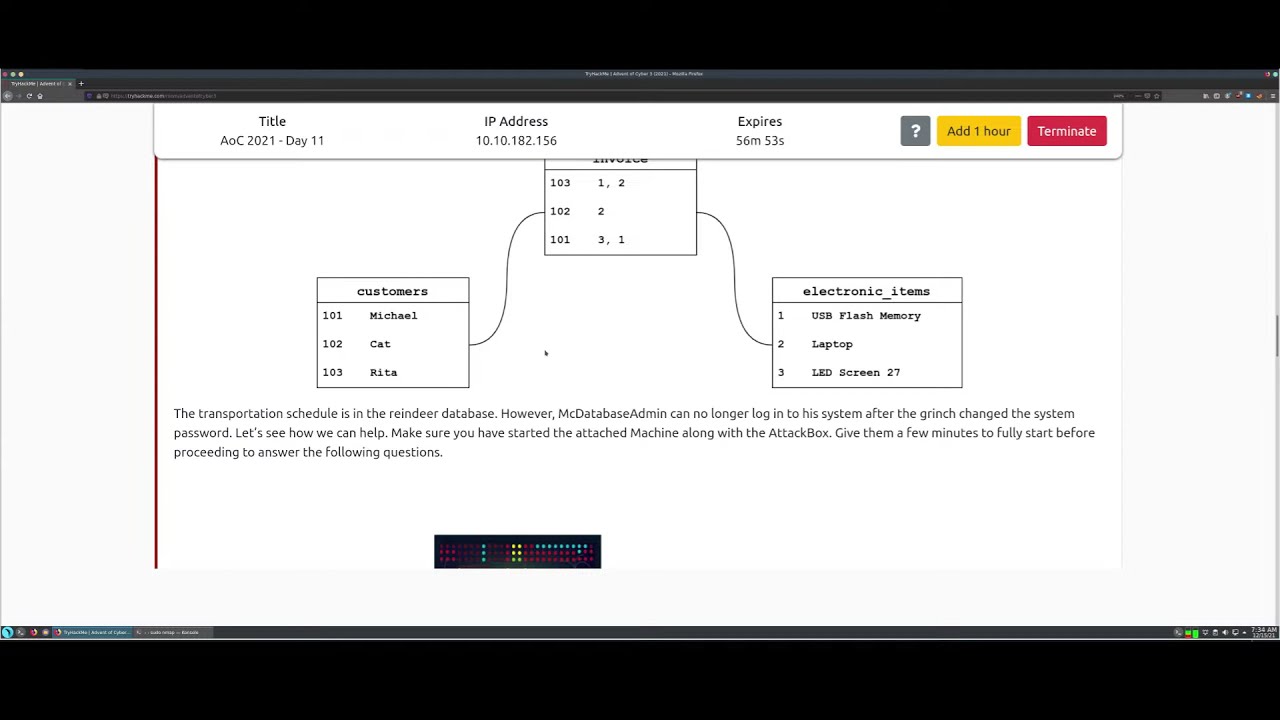This image appears to be a screenshot of a web page, possibly related to a puzzle or task management system. The web page has a black thick border along the top and bottom, with a white center section. At the very bottom, there's a thin black line with white borders, containing text and shapes.

At the center of the white area, there's a prominent section marked out in black and red. In black text, it reads: "Title: AOC 2 2021 Day 11, IP Address: 10.10.182.156, Expires: 56 minutes 53 seconds." Adjacent to this text, there's a small black box with a white question mark, a yellow tab labeled "Add one hour," and a red tab labeled "Terminate."

Just below this section, there are three black-framed squares. Each square contains different information, such as "Customers" and "Electronic Items," with respective numbers and other text inside them. The squares are interconnected by squiggly lines forming an S-shape and backward X-shape, linking box to box.

Beneath these connected squares, there is a block of black text explaining a problem regarding the transportation schedule being stored in a reindeer database and mentioning the McDatabase administration's inability to log in after the system password was altered by the Grinch. The text suggests solutions and prompts to start the attached machine and attack box, followed by additional instructions or questions.

At the very bottom of the image, there’s a black rectangular area with text in different colors—red, blue, and yellow—providing further details or prompts.